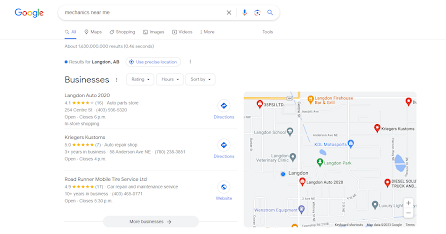In the image, a Google search is displayed on a computer screen with the query "mechanics near me." The search results page shows tabs for different categories such as All, Maps, Shopping, Images, Videos, and More. The page also indicates the total number of results and the time taken to generate them.

Prominent businesses appear in the search results:

1. **Langdon Auto**: Rated 4.1 stars, this business is currently open and closes at 6 p.m. The listing provides a phone number and a blue "Directions" button on the right.

2. **Krieger's**: This mechanic business boasts a perfect 5.0-star rating with stars highlighted in yellow. It mentions being in business for over three years, provides their phone number, and states that they are open until 4 p.m. The listing also features a blue "Directions" button.

3. **Roadrunner Mobile Towing Service LTD**: Holding a 4.5-star rating, this service also includes a clickable "Directions" button.

A map is visible on the right side of the screen, marked with pins indicating the locations of these businesses.